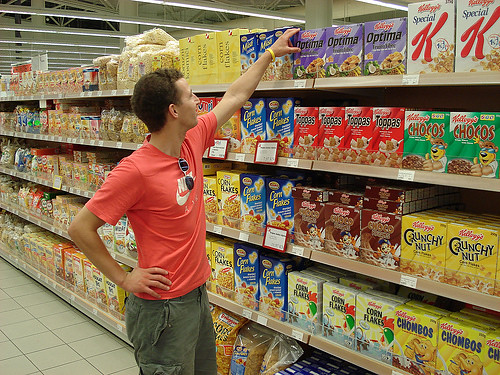In the bustling cereal aisle of a grocery store, a man wearing a red Nike shirt with aviator-style sunglasses hanging from the neckline stands thoughtfully. With one hand on his hip and the other reaching out, he appears on the verge of selecting a box of Kellogg's Optima cereal. The shelves around him are a colorful array of breakfast options, including a neighboring, yet indiscernible, blue cereal box, Special K to the opposite side, and below it a mix of cereals like Cornflakes, Froot Loops, and Kellogg's Chocos. Dressed in Army green cargo shorts, he seems to be weighing his options, likely favoring the Optima cereal but still contemplating his choice.